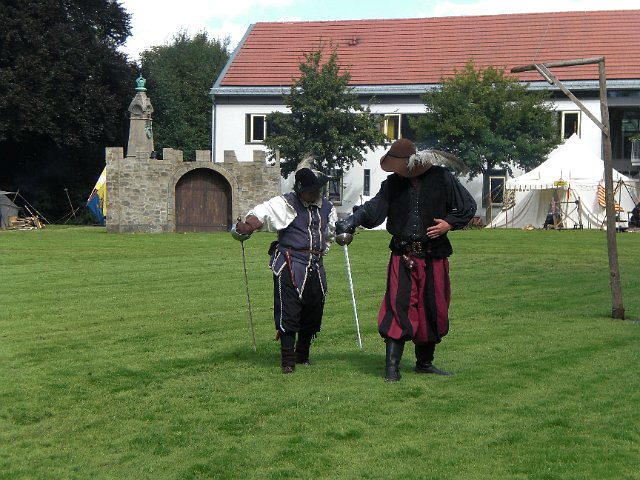In this photograph, two individuals dressed in Renaissance fair attire stand on a well-manicured, green lawn. The person on the left is attired in a white long-sleeve shirt with a blue vest, black pantaloons, and black boots, topped off with a black hat adorned with a plume. They are holding a saber in their right hand, facing slightly forward and right. To their right, another person is dressed in a dark-colored shirt with a black vest, purplish pantaloons with black vertical stripes, and black boots, donning a brown wide-brimmed hat also featuring a feather. This person holds a saber in their right hand, extending it to the left. In the background, a white-painted, two-story building with a red roof is visible. To the left of this building, there is a small structure resembling a castle entrance with a stone facade, two arched doors, and a steeple. Slightly to the right of the individuals, a white triangular tent supported by wooden poles stands out against the open sky. Adjacent to the tent, a wooden post with a crossbar is also noticeable. Further details include trees and wooden materials to the left of the castle-like structure, enhancing the scene's historical ambiance.